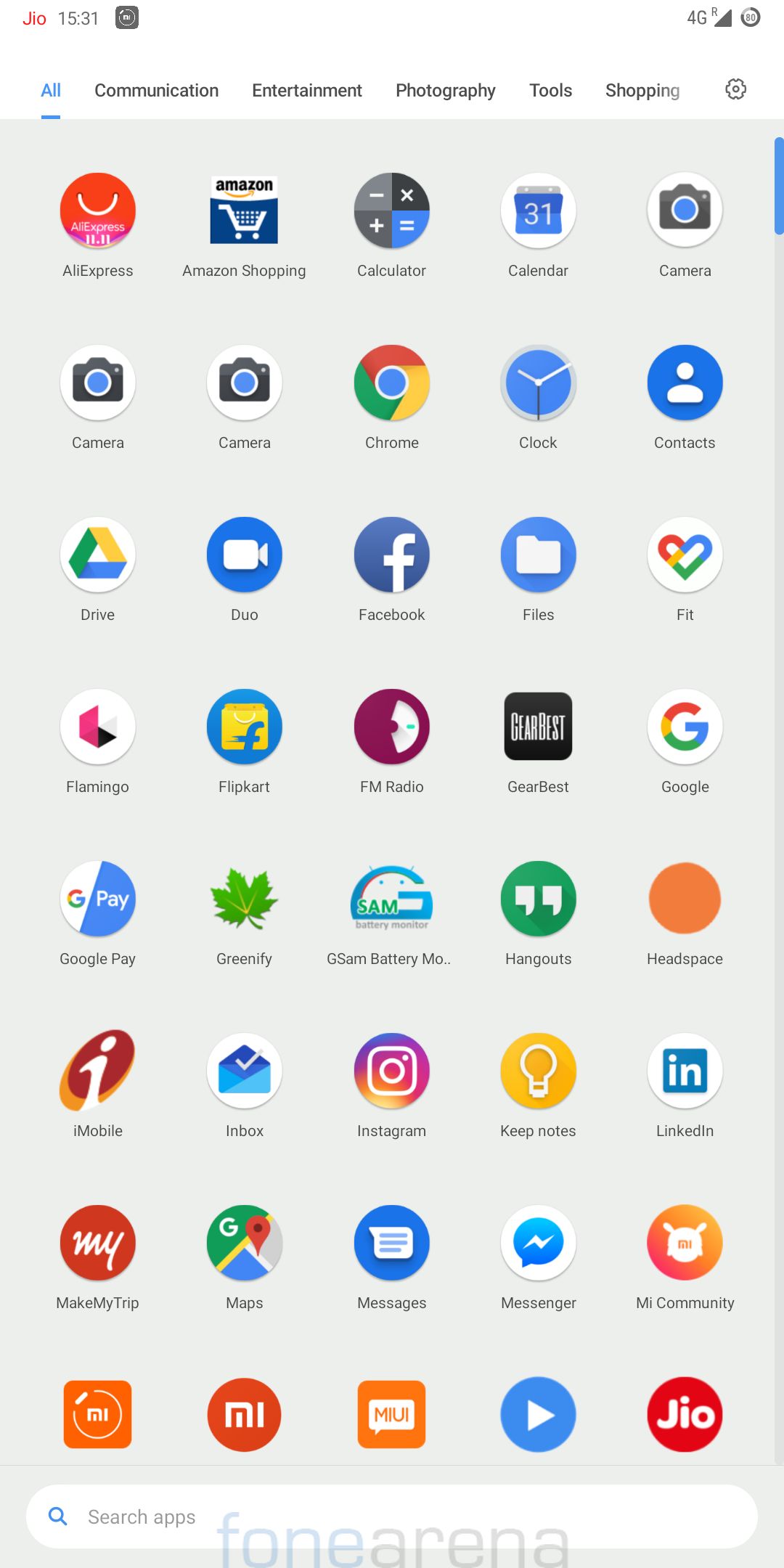Here's a detailed descriptive caption based on your input:

---

The image features a digital screen, likely a tablet or a large smartphone, with the "JIO" logo in red text displayed at the top-left corner. The status bar indicates the time as 15:31 (3:31 PM), alongside icons for 4G connectivity, a right-pointing triangle with an 'R' above it, and several undiscernible symbols.

Central to the screen is a navigational menu with categories such as Communication, Entertainment, Photography, Tools, Shopping, and Settings. The 'All' category is currently selected, highlighted in blue text with an underline, while the other categories remain in black text.

Below the menu, multiple app icons are displayed in circular frames, with a few exceptions detailed later. The visible icons include:

- **Aliexpress:** Red background with the Aliexpress logo.
- **Amazon Shopping:** Blue background with the Amazon shopping logo.
- **Calculator:** Symbolized by mathematical operators (minus, plus, times, equals).
- **Calendar:** Classic calendar icon showing the number 31.
- **Camera:** Three instances, each displaying a camera icon.
- **Chrome:** Multi-colored circle with blue, red, yellow, and green segments.
- **Clock:** Traditional clock icon.
- **Contacts:** Silhouette of a person inside a circle.
- **Google Drive:** Yellow, blue, and green ribbon forming a triangle inside a circle.
- **Duo:** Video camera icon in blue.
- **Facebook:** White 'F' on a blue circle.
- **Files:** Blue circle with a file folder icon.
- **Fit:** Heart-shaped icon with colors from the Google logo, likely Google Fit.
- **Flamingo:** Pink and white icon of a flamingo.
- **Flipkart:** Yellow shopping bag with a blue 'F' appearing to move.
- **FM Radio:** Symbolized by a half-circle with a blue line.
- **Gearbest:** Exceptionally not in a circle, a black box with "Gearbest" text.
- **GSAM Battery Monitor:** A stylized 'G' resembling a battery gauge.
- **Greenify:** Depicted by a leaf.
- **Google:** Multi-colored 'G' within a circle.
- **Google Pay:** Circle divided into blue and white segments with "G Pay" text.
- **Hangouts:** Green circle with parentheses.
- **Headspace:** Entirely orange icon.
- **iMobile:** Red and orange circle with a white 'i'.
- **Inbox:** Envelope with a white checkmark.
- **Instagram:** Camera icon with a gradient of pink, purple, and yellow.
- **Keep Notes:** Yellow circle with a white light bulb.
- **LinkedIn:** Blue square with 'in' text inside a white circle.
- **Make My Trip:** Red circle with 'my' text.
- **Google Maps:** Icon of maps with a location pin within a circle.
- **Messages:** Blue circle with a white speech bubble.
- **Messenger:** White circle with a blue speech bubble featuring a lightning bolt.
- **Me Community:** Orange circle with an icon.
- **Mi Apps:** Not fully readable, featuring multiple "mi" labels.
- **Play Store:** The traditional Play Store triangle icon.
- **Jio:** Icon with the JIO logo.

Additional on-screen text prompts the user to "Search apps," and there's a watermark reading "PhoneArena" in the background.

---

This structured and detailed description captures all the elements described in the original spoken input, organizing them systematically for clarity.